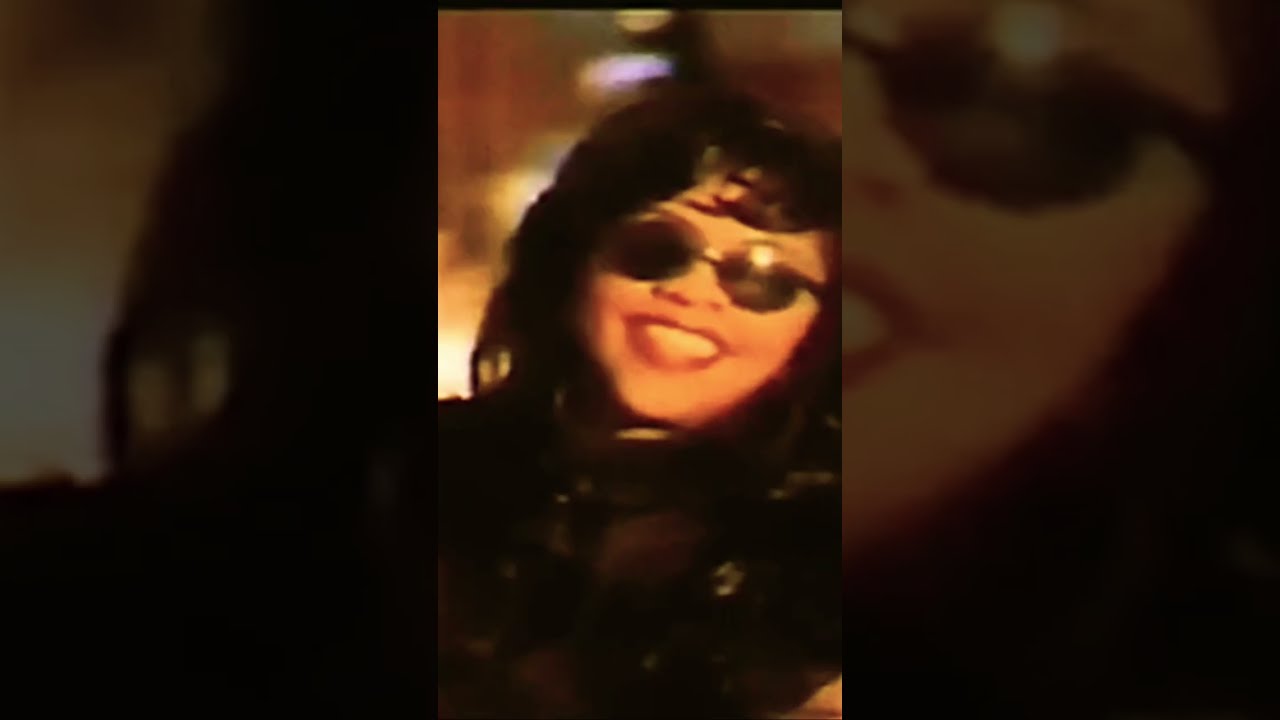The photograph features a young African-American woman, likely a singer in her mid-twenties, with a big smile revealing her white teeth. She has shoulder-length, dark brown to black hair, with bangs swooping to one side. She is wearing round, dark sunglasses that reflect a circle of light off the top right of the right lens. Her nose is slightly flared, and her lips are bright red. The image has a soft, noisy texture suggesting it might be from an older video, with dim, blurred lights in the background hinting at a nighttime cityscape. She is dressed in dark clothing that appears to have a pantyhose-like texture, possibly a black bra under a semi-transparent top. The photograph itself is vertically cropped and features an expanded, blurred-out version of her face in a rectangular border, giving the entire image a layered effect.